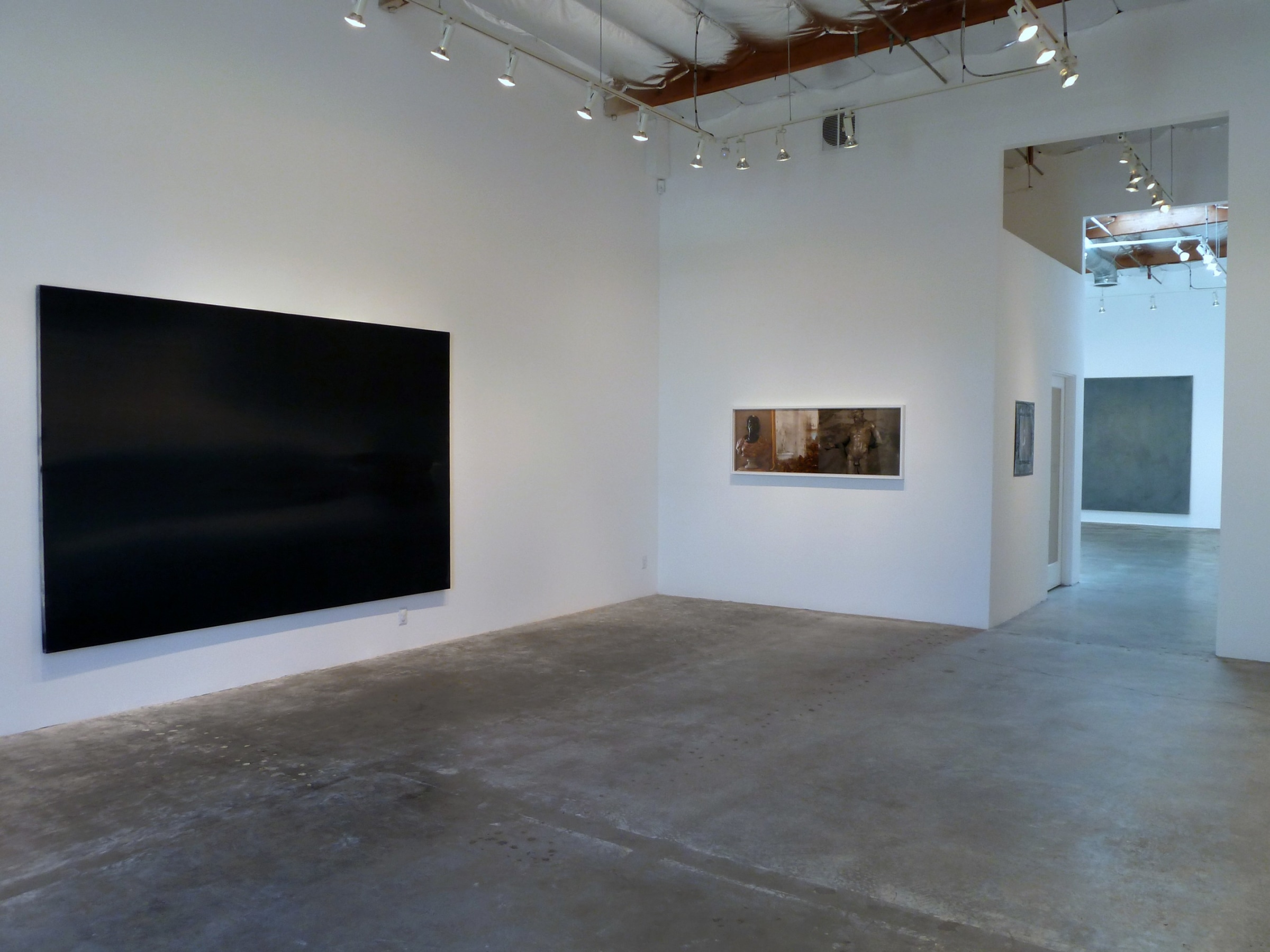The photograph showcases the interior of an industrial-looking building taken in landscape mode. The room captured appears unfinished, with dark gray concrete floors featuring brown and black spots that run across the bottom third of the image. The walls are stark white, and overhead lighting is structured in rows forming a square, with the fixtures emerging from a dark wood box accentuated by white tubes. 

A large black monitor is mounted on the left wall, positioned above an electric socket. Adjacent to this, the top center reveals exposed ductwork likely serving heating and cooling purposes, surrounded by numerous floodlights. 

On another wall, there's a painting featuring greens, reds, and browns, contributing a touch of color to the otherwise monochromatic space. The room extends into a hallway leading to another section of the building, which might be a secondary room. It contains what appears to be a painting resembling a giant chalkboard. The floor, consistent with the hall’s industrial theme, displays seams indicative of being pieced together or patched. This secondary room is also adorned with additional floodlights similar to those in the main area. The overall ambiance suggests a place not currently in use or perhaps under construction, characterized by its raw, unfinished aesthetic.